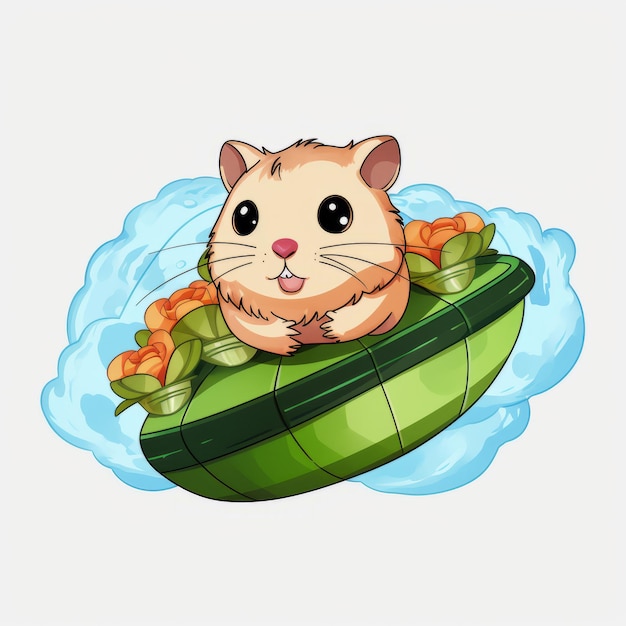This illustration features a charming hamster with round black eyes reflecting light, a cute pink nose, and a slightly open mouth, emphasizing its adorable nature. The hamster, with its intricately detailed brown and tan fur, is depicted sitting in a green, UFO-like bowl. The bowl, which could be interpreted as a levitation device or spaceship, has a dark green center band and is adorned with orange flowers sprouting from green plants. Blue clouds or cloud-like smoke trail behind the spaceship, implying movement. The background is a light gray, further highlighting the hamster and its unique floral spaceship, which appears to be flying or floating in mid-air, reminiscent of Japanese anime style. The composition is set on a white backdrop, drawing focus to the whimsical scene.